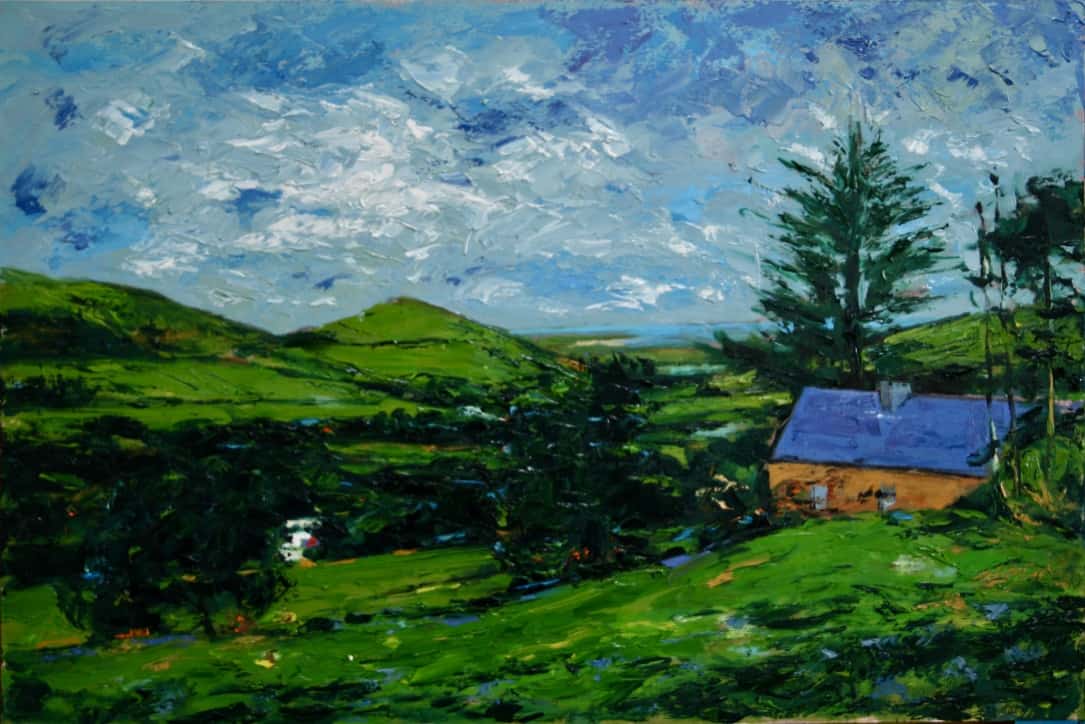This oil painting depicts a vibrant and idyllic outdoor scene characterized by rolling, lush green hills dotted with an array of trees and wildflowers. In the foreground, a small house with a royal blue roof, a chimney, and rustic orange walls nestles comfortably amidst the verdant landscape. The grassy terrain is interspersed with hues of light orange, blue, and red, indicative of wildflowers thriving in the area. A person is visible outside on one of the hills, adding a touch of human presence to the natural setting. The sky above features a mix of light clouds and deeper, dark gray ones, while faint white clouds add depth to the blue expanse. In the background, additional houses and perhaps a glimpse of a distant body of water can be seen, partially obscured by the undulating hills and scattered pine trees. The scene is further animated by what appears to be colorful butterflies fluttering around, enhancing the overall tranquility and beauty of the landscape.